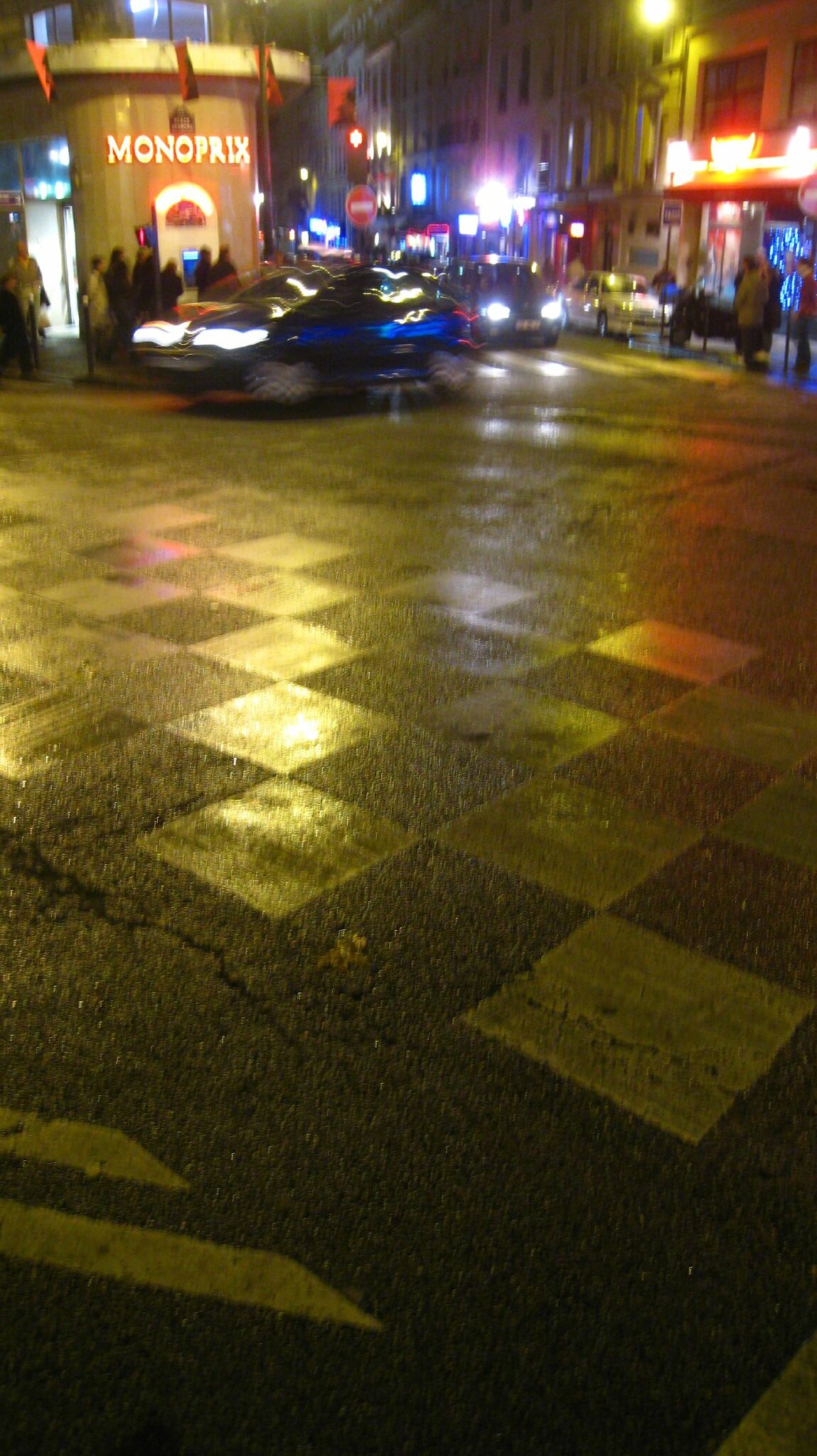The photograph captures a bustling European city street at night, taken in portrait mode with a long exposure, which gives the lights a soft, blurred effect. The foreground features a checkerboard-patterned pavement leading towards the street, where cars, with their headlights on, can be seen driving through the scene. On the other side of the street, numerous people are gathered, appearing as blurred figures due to the long exposure. Prominently displayed on a building to the left is a Monoprix sign illuminated in red LED lights, adding to the nighttime urban ambiance. Additional neon signs and a red traffic light further accentuate the vivid scene. Buildings with both illuminated and dark windows form the background, providing depth and context to this visually dynamic urban nightscape.